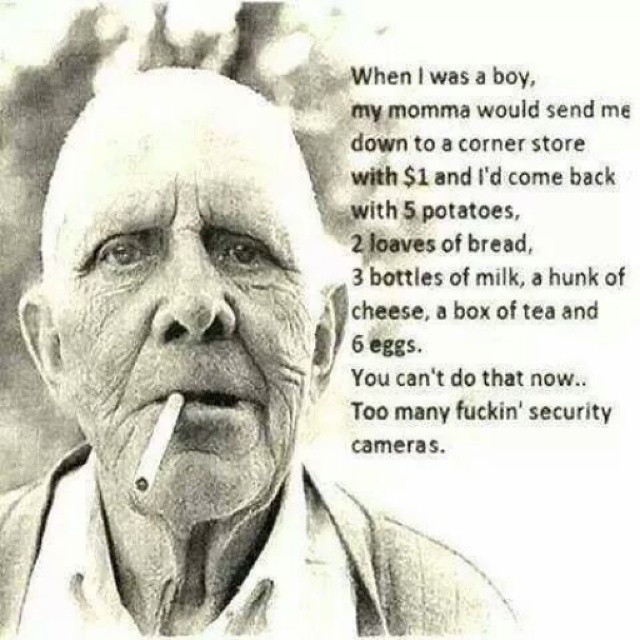The photograph captures an elderly, bald man with deeply wrinkled skin and a serious expression. He is wearing a collared shirt under a sweater or jacket. The image is in black and white or sepia tone, characterized by shades of white and tan. A cigarette dangles from the corner of his mouth. The background is hazy with a grayish tone and subtle shadows, possibly resembling a tree against the sky. To the right of the man's profile, written in black text, is the quote: "When I was a boy, Mama would send me down to a corner store with a dollar and I'd come back with five potatoes, two loaves of bread, three bottles of milk, a hunk of cheese, a box of tea, and six eggs. You can't do that now. Too many fucking security cameras."